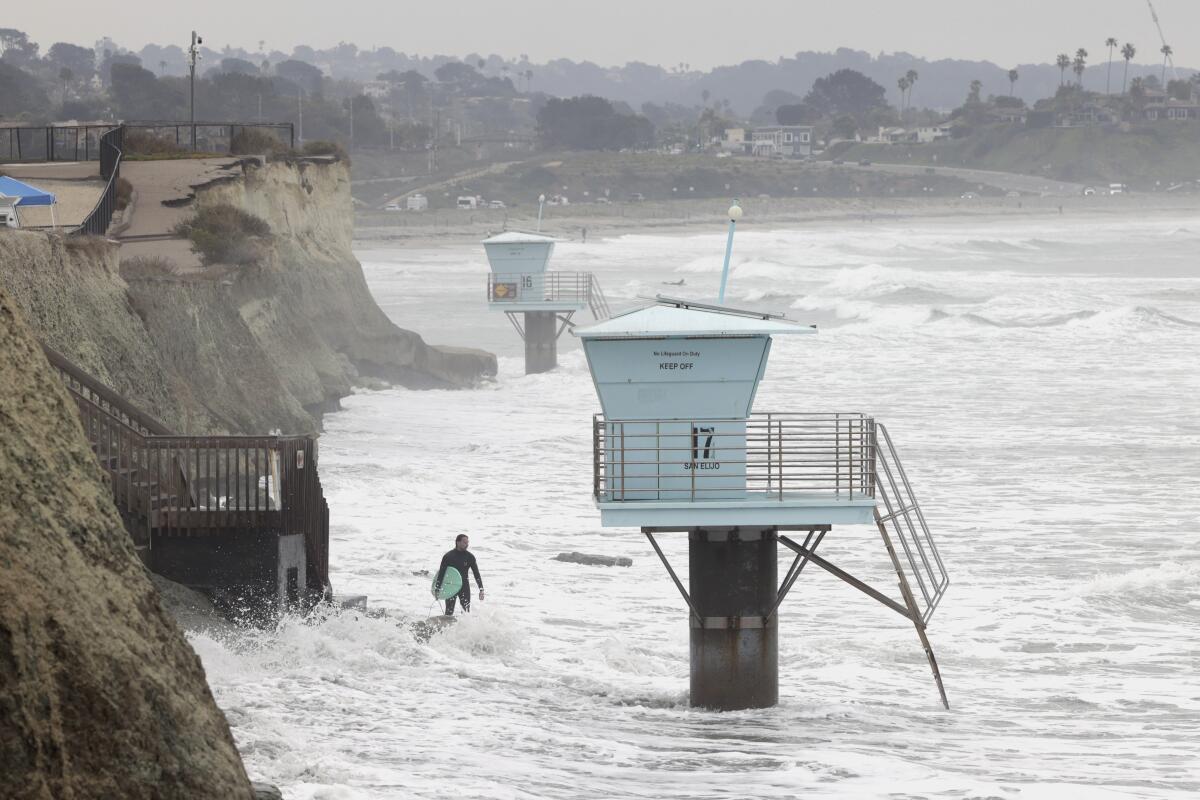In this detailed outdoor image captured in daylight, the scene prominently features a vast expanse of ocean with dynamic waves and white caps. The backdrop showcases distant hills, trees, and a field, lending a scenic quality to the horizon. On the left side of the image, a steep, rocky wall extends from the bottom left to the upper left, featuring jagged concrete remnants as though a road once traversed it but has since collapsed. Nestled against this rocky outcropping is a wooden staircase that descends to the water level, leading to a beach area now completely inundated with water, leaving no visible sand.

Two lifeguard towers with distinctive cement pillars and small white cabins, each having a metal walkway around them, stand amidst the water. At the base of one of these towers, a man in a black wetsuit stands in the ocean, holding a surfboard. The entire beach area appears to have suffered significant erosion and flooding. Adjacent to the left side, another set of stairs is attached to a hill adorned with barricades, a viewpoint, and sitting areas at the top, offering a vantage point over the tumultuous waters.